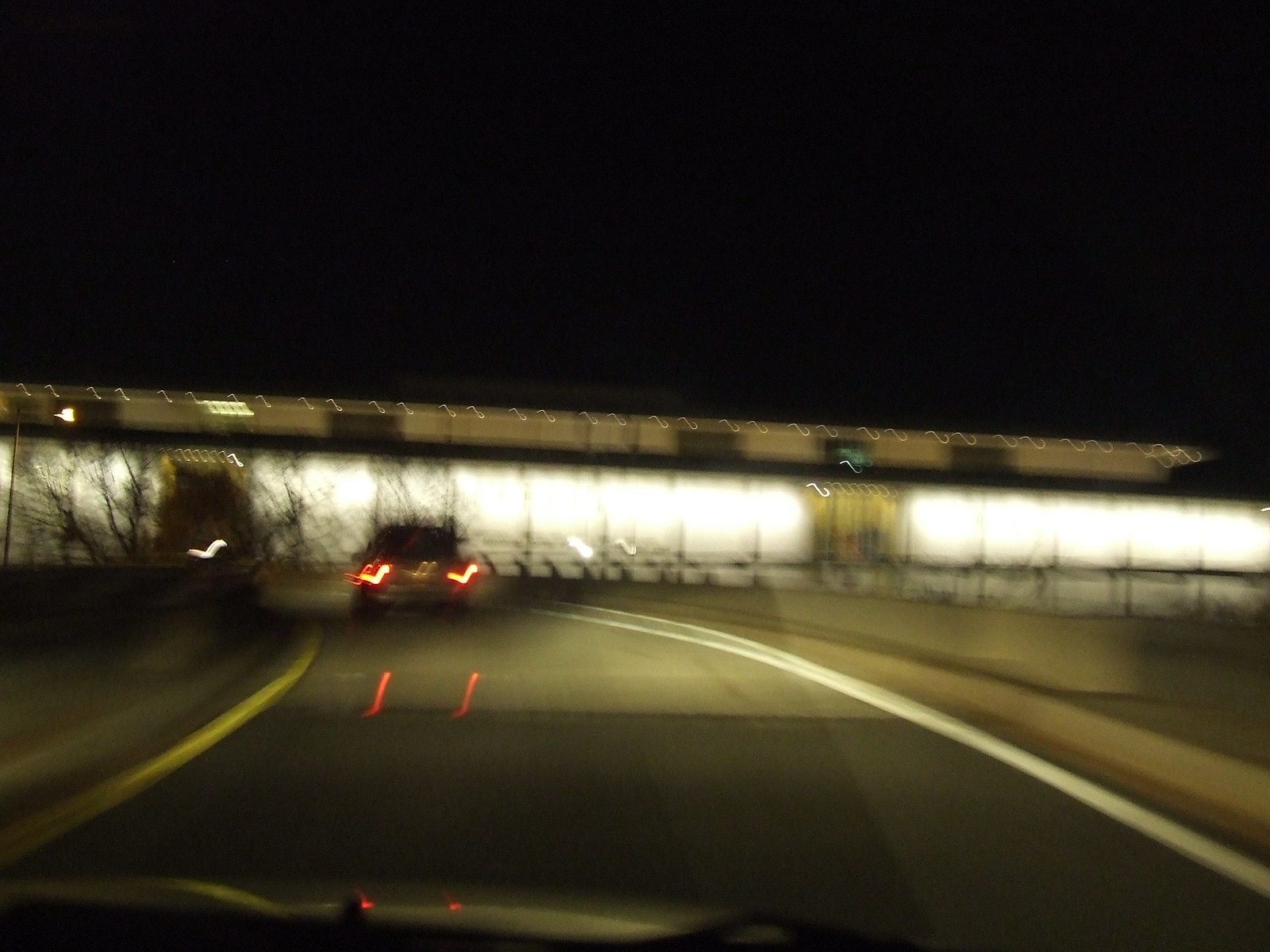This image is a blurry, horizontally oriented, color snapshot photograph taken from the driver's seat of a car, looking out through the windshield as the vehicle is navigating a left-hand turn. A narrow yellow stripe is visible along the left quarter of the image, emphasizing the curve of the road, while a broad white stripe marks the road's edge in the bottom right corner, extending towards the center. Prominently featured across the horizon of the image, a row of illuminated rectangles suggests the presence of a toll booth or building adjacent to the road. Bright lights emanate from this structure, casting a pale glow over the scene. In front of the viewer, the taillights of a car turning the same corner are visible, creating a distinctive V shape on the windshield that highlights the vehicle's movement.